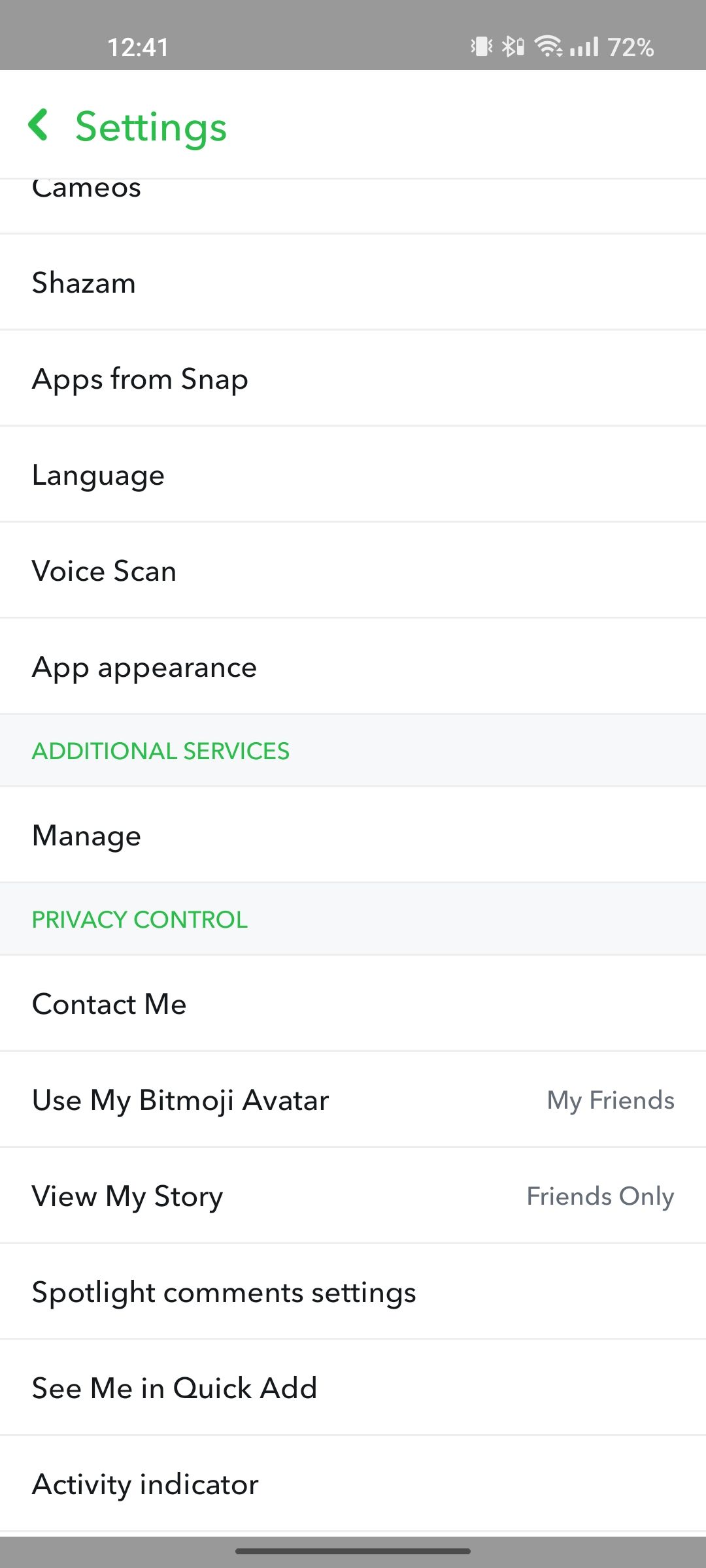This screenshot captures an image of a smartphone screen. At the top of the screen, a gray notification bar displays the time "12:41" on the left side, while the right side shows icons for Wi-Fi connectivity, full cellular reception, and a battery level at 72%. Directly below, on a white background, the word "Settings" is prominently displayed in bold green text. 

The menu detailed beneath "Settings" includes various options listed vertically:

1. Cameos
2. Shazam
3. Apps from Snap
4. Language
5. Voice Scan
6. App Appearance

A secondary section, titled "Additional Services" in green text, appears below these options, followed by the item "Manage."

Further down, the "Privacy Control" section includes the following:

1. Contact Me
2. Use My Bitmoji Avatar
3. View My Story
4. Spotlight Comments Setting
5. See Me in Quick Add
6. Activity Indicator

Separating these sections is a gray horizontal divider with a small horizontal black line in the center, enhancing the visual clarity of the screen layout.